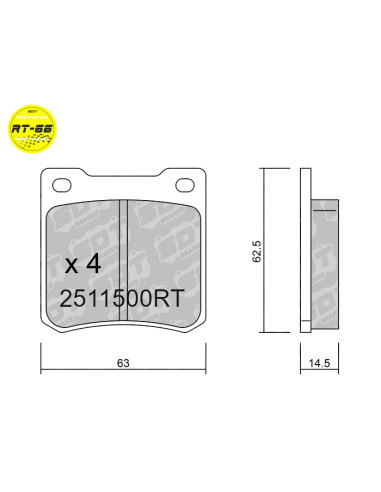The image is a black-and-white technical line drawing in landscape orientation. On the left side, it features a yellow circle with the text "RT 66." Below the circle, there is a rectangular shape with two holes on either side, possibly for handles. In the center of this rectangle, there is a gray section displaying the text "X4 2 5 1 1 5 0 0 RT." At the bottom of the rectangle is a measuring scale marked "63." To the right of the rectangle, there are additional measuring details with "62.5" and "14.5" marked on cylindrical shapes. The background is white, giving the drawing an impression of a product specification sheet or a technical diagram, possibly related to automotive parts.